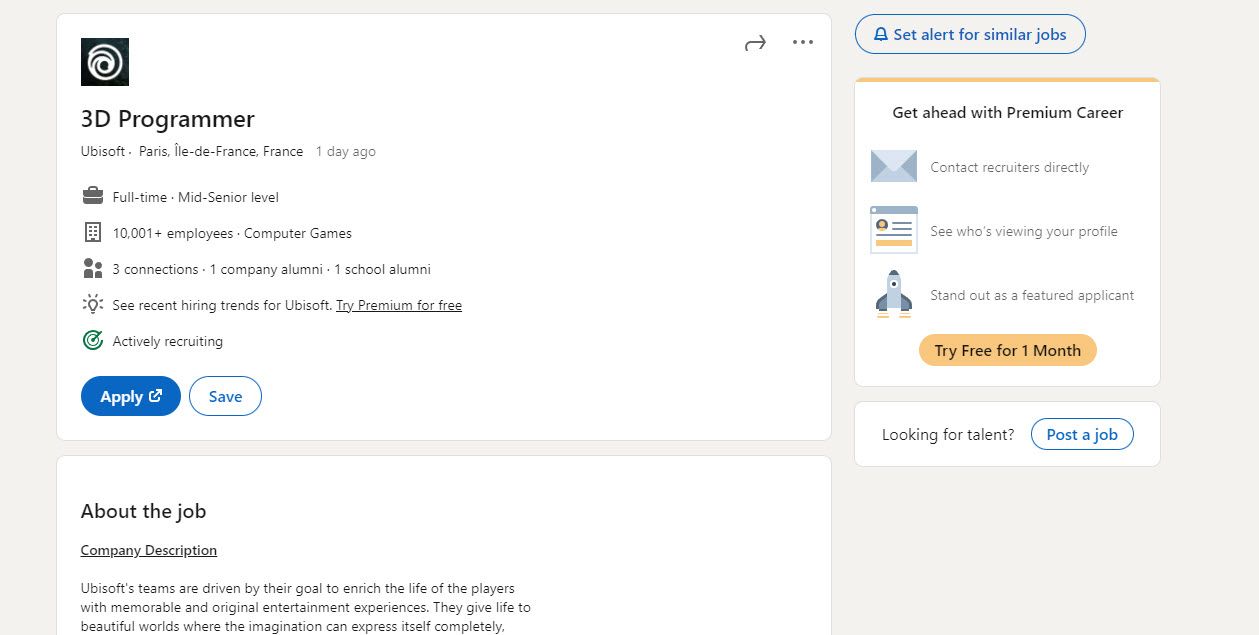**Detailed Caption:**

The screenshot depicts a job listing interface on a light beige background. On the left side, there are two prominent white rectangular sections with detailed job information. 

The upper section includes a black icon at the top, denoting the position of "3D Programmer," followed by a note that indicates the job location is in France and it was posted one day ago. Several small icons provide additional details:
- A full-time job status icon,
- A company size indicator showing 10,000 employees,
- A person icon indicating three current connections within the company,
- A light bulb icon displaying a prompt to "See recent hiring trends,"
- A recruitment status icon showing "Actively Recruiting."

Beneath this, there are two buttons: a blue button with white text labeled "Apply," and a second button with a white background and blue outline, labeled "Save."

The section continues with a job description and details about the company. Additionally, on the upper right corner of this section, there is an arrow and a three-dot menu for more options.

To the right of the job listing, there's a button with a gradient light blue to dark blue line and an alarm icon, labeled "Set alarm for similar jobs" to enable notifications for similar opportunities.

Below this, there's another white square with a yellow top border. This section promotes a premium career service with the headline "Get ahead with premium career" and mentions a trial offer, "Try free for one month," flanked by an envelope and paper bracket icons.

At the bottom of the interface, there's an invitation to "Post a job" for those seeking talent.